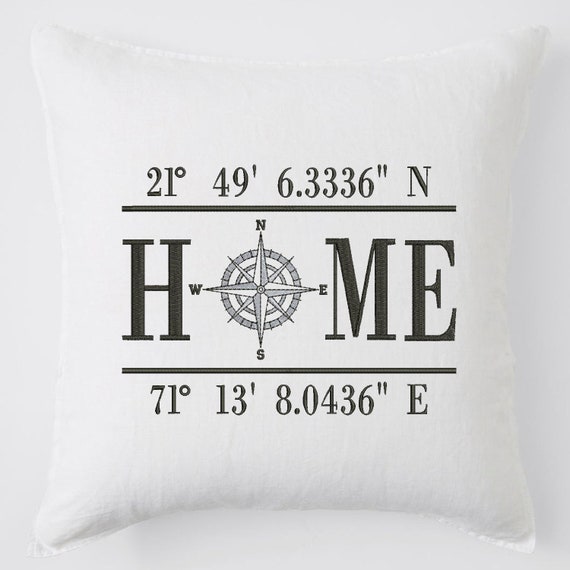This is a detailed photograph of a square-shaped pillow that is white with a black and gray design, set against a light gray background. The pillow subtly curves inwards on each side. Prominently in the center, the pillow features the word "HOME" in large black capital letters, where the "O" is artistically designed as a compass displaying cardinal directions (N, S, E, W). Above the word "HOME," the pillow shows precise geographical coordinates: "21° 49' 6.3336\" N", with a black horizontal line beneath it. Below the word "HOME," another set of coordinates is displayed: "71° 13' 8.0436\" E", also underscored by a black horizontal line. These coordinates are meticulously detailed with degrees symbol, apostrophes, and quotation marks to denote minutes and seconds.